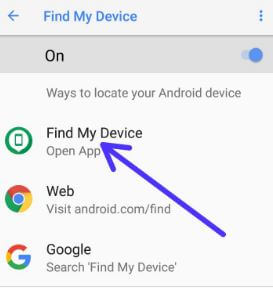The image is a square with a grayed-out background. At the top, prominently displayed, is the text "Find My Device" with a left-pointing arrow next to it, indicating a breadcrumb navigation element showing the user has selected this option. On the far right of this header are three vertically aligned dots, suggesting additional settings or options.

Below this header, there is a slightly darker gray rectangle with the word "On" in black text, accompanied by a blue toggle button set to the "On" position. 

Underneath this, centered within the box, the text reads "Ways to locate your Android device" in a lighter gray font. 

Following a couple of spaces, the next section features the option "Find My Device" in darker black text. Just beneath that, "Open App" is displayed in gray, accompanied by a green circular icon featuring a phone image at its center.

The next option is "Web," which displays the Google Chrome logo and the URL "visit android.com/find."

The final option in this section is represented by a Google logo with the text "Search 'Find My Device'" in quotation marks.

A large bluish-purple arrow emanates from the bottom right corner of the image, pointing upwards towards the "Find My Device" heading, drawing attention to this primary feature.